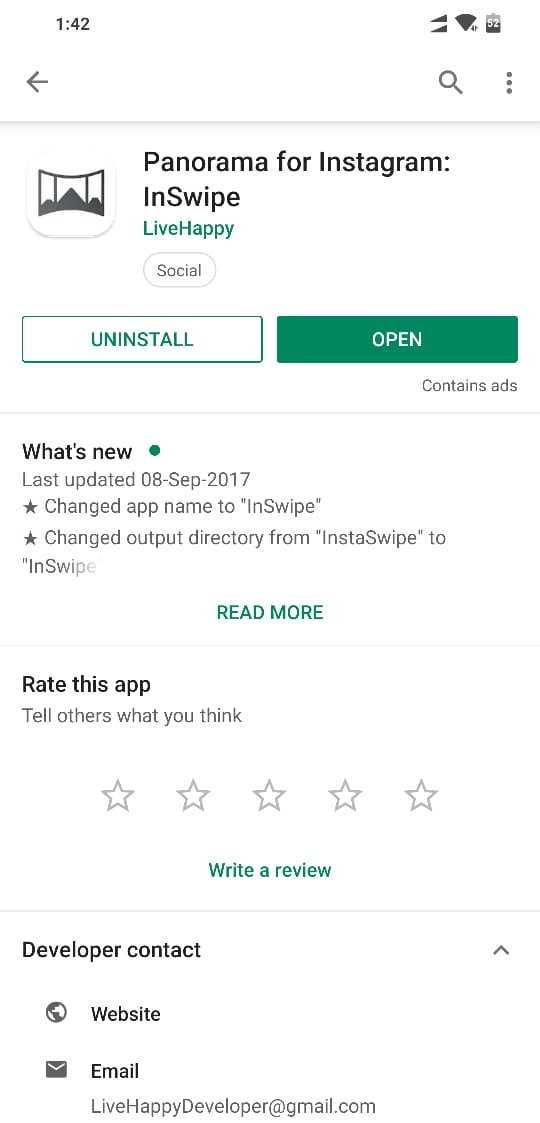The image depicts a settings section for a mobile application on a device. The device displays the time as 1:42 in the upper left corner, with the battery level at 52%. Below the time and battery indicators, there are a back arrow and a search icon. The application being viewed is "Panorama for Instagram InSwipe" by Live Happy, categorized under "Social."

Prominent buttons include "Uninstall" and "Open" for managing the app. Information about the app’s latest update is provided, stating it was last updated on September 8, 2017. The update details include a change in the app name to "InSwipe" and a modification of the output directory name from "InstaSwipe" to "InSwipe," with a "Read more" option for additional details.

Users are encouraged to rate the app via a five-star rating system and have the option to write a review. Developer contact information is provided, including options to visit the developer's website or send an email, with the email address displayed for convenience.